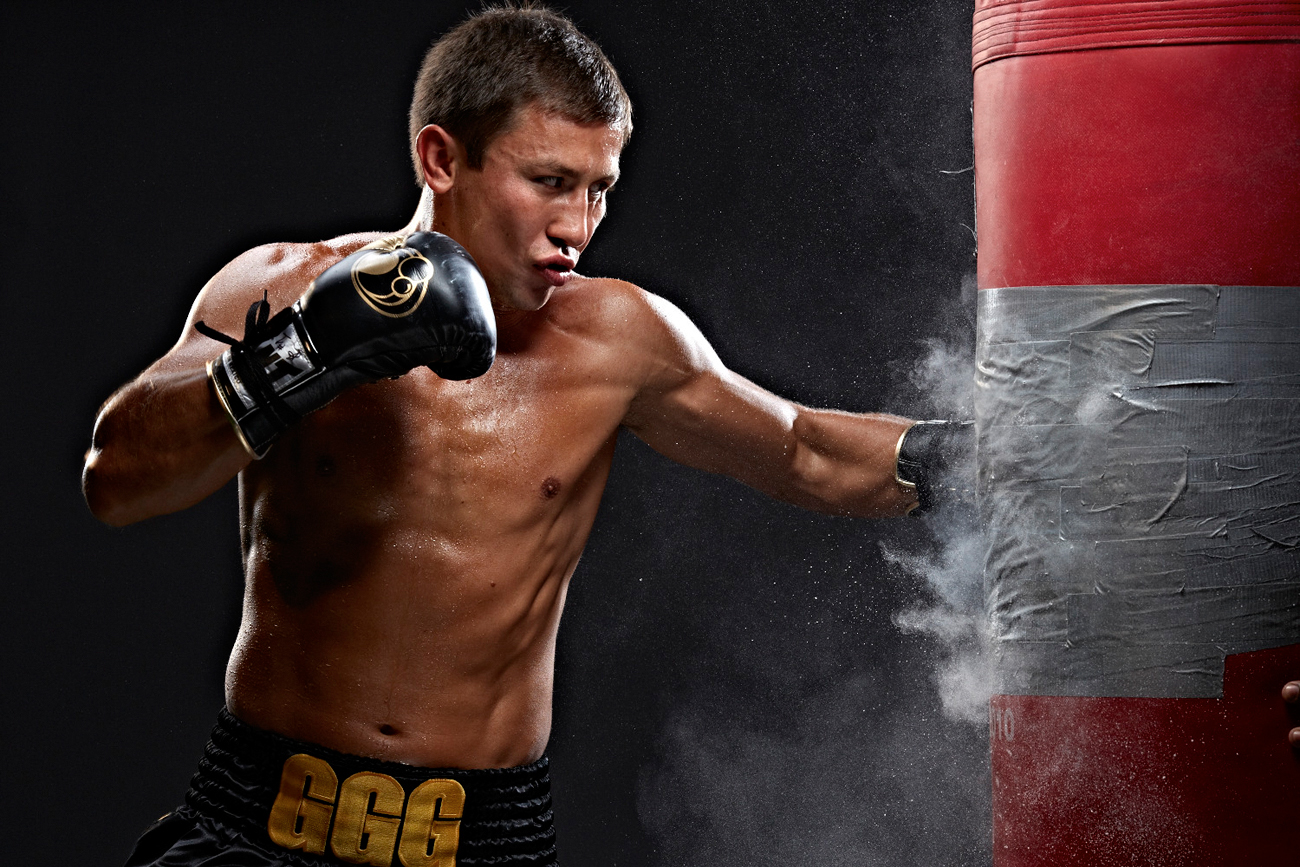This dynamic action shot captures a shirtless, sweaty boxer of apparent Asian descent, intensely focused on his training as he delivers powerful punches to a duct-taped red punching bag, causing a cloud of white chalk or dust to explode from the bag with each impact. The boxer, seemingly in his late 20s and sporting a deep tan, wears intricate black boxing gloves with gold emblems and sleek black boxing shorts featuring a wide waistband emblazoned with the gold letters "GGG." His facial expression, with pursed lips, reveals his deep concentration and dedication, making this image ideal for a promotional advertisement or an upcoming fight brochure.